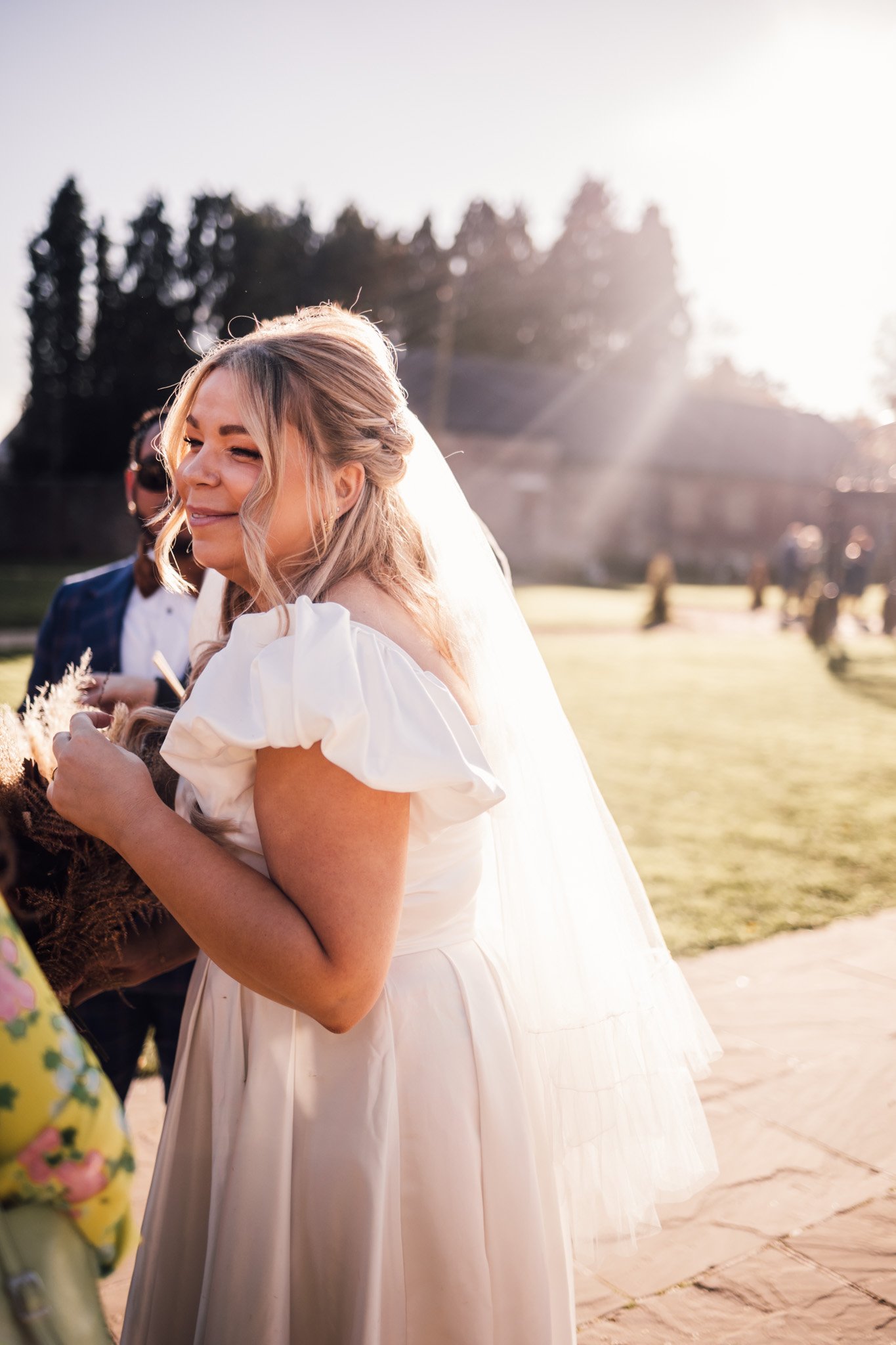In this vertical, rectangular color photo, a bride and a partially visible man are captured outdoors on a bright, sunny day. The woman, positioned on the left side of the image, is wearing a white wedding gown with very short puffy sleeves and a long veil that extends past her waist. Her dirty blonde hair features wisps along the sides of her face and she appears to be either squinting or shutting her eyes as she looks to the side, away from the sun which shines brightly in the top right corner of the image. 

Adjacent to her, the man is seen with his face partially visible, adorned in sunglasses, a blue suit, white shirt, and a bow tie. They both stand on a stone walkway with a backdrop that includes a field of grass and a large building, which is exceeded in height by tall trees. The top of the image reveals a clear view of the sky, blending seamlessly with the sprawling trees and the blurred elements in the background.